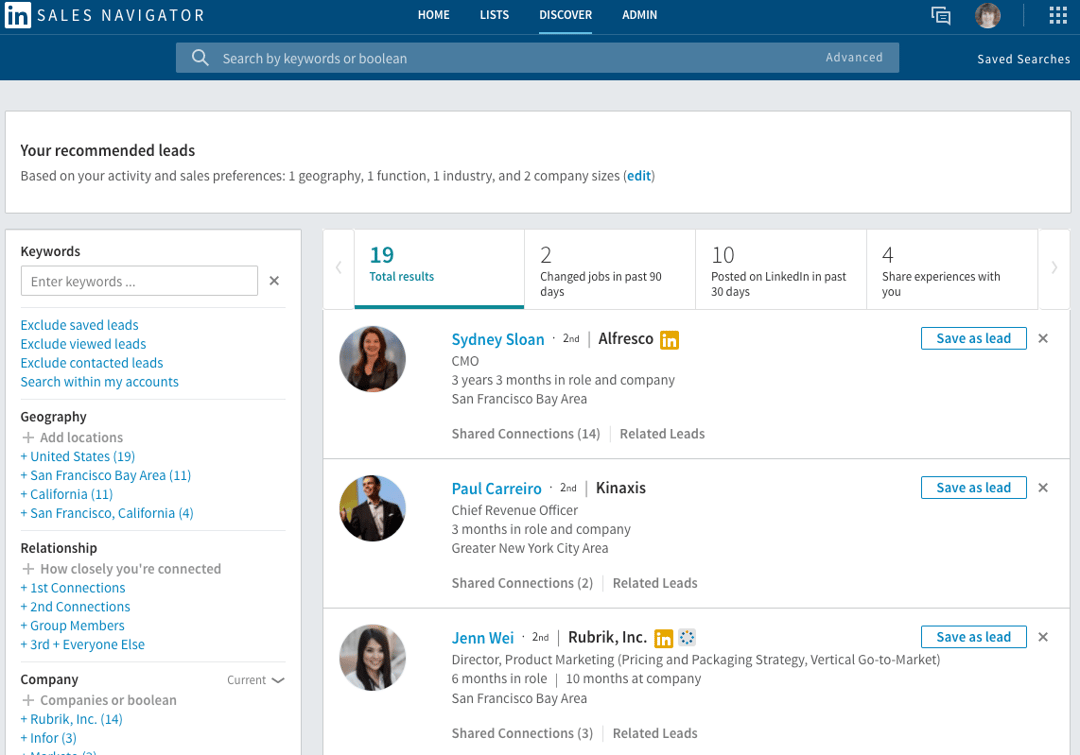**Detailed LinkedIn Sales Navigator Screenshot Description:**

This image is a screenshot of the LinkedIn Sales Navigator interface. In the upper left corner, the IAM logo is visible, with the text "Sales Navigator" displayed to its right. The top navigation bar features options such as Home, Lists, Discover, and Admin in the center. On the right side of this bar, there are several icons including a grid menu, profile photo, speech bubbles, and a save searches option.

Dominating the center of the interface is a large, light blue search bar that reads "Search by keywords or boolean." Below this search bar is a gray field with a white rectangular overlay, indicating "Your recommended leads based on your activity and sales preferences." It lists filters like geography, function, industry, and company sizes, with an option to edit this criteria, marked in blue within gray brackets.

On the left side of the screen, a vertical menu offers various search filters. It starts with "Keywords," allowing users to enter search terms and include or exclude certain criteria. Below this, there are three more sections: Geography, Relationship, and Company, each with blue options like locations (e.g., United States, San Francisco), relationship types (e.g., first connections, second connections), and company names as relevant filters.

To the right of the filters, there are displayed results, summarizing the search output: "19 total results" highlighted in blue, alongside "2 changed jobs in the past 90 days," "10 posted on LinkedIn in the past 30 days," and "4 shared experiences with you," all in gray text.

The screenshot shows three specific individuals: Sidney Sloan, Paul Correrio, and Jen Wei. Each name is accompanied by a circular photo on the left, their current positions—CMO, Chief Revenue Officer, and Director of Product Marketing respectively—and a "Save as lead" button on the right for each individual.